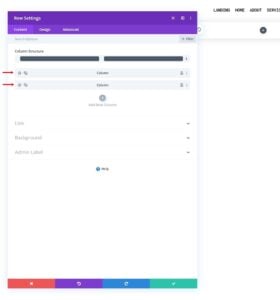A screenshot of a settings page displayed on a mobile device or tablet featuring a vertically-oriented layout. The top of the screen showcases a purple banner that reads "Settings" and possibly "New Settings," with both a close button and a more options button visible. In the upper right corner, "Home" and "About" are listed as additional clickable options. The image includes multiple colors such as purple, red, blue, and green, but it is difficult to discern specific details due to the low resolution and small size. The summary section beneath the banner is particularly unclear; it consists of two dark gray lines and two thinner gray lines, each highlighted with red arrows. Below these lines, there are three pieces of information that are unreadable due to the image quality.